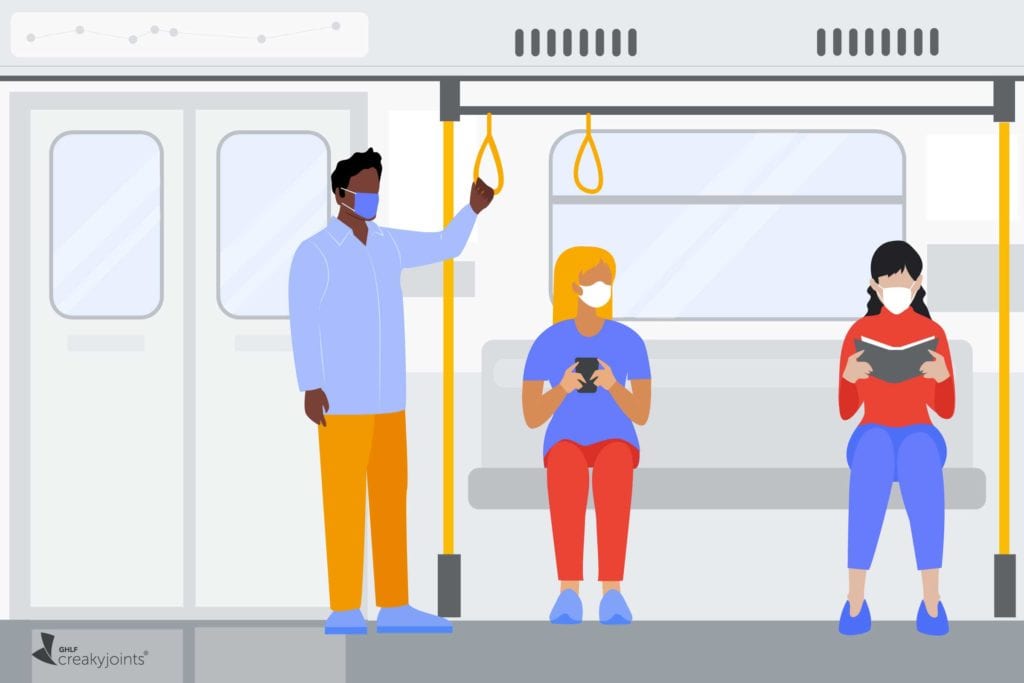This detailed infographic, rendered in a generic, corporate art style typically used for public service announcements, depicts a scene inside a subway train. The simplistic, shapeless blob-like characters lack intricate facial details, yet distinctively highlight their activities and attire. The background features elements like the subway door, window, light grey bench, white walls, and dark grey floor. Standing in the middle is a black man wearing a blue long-sleeve shirt, orange (or yellow) pants, and a blue face mask, holding onto a yellow handle. Seated on the bench are two women, both donning face masks. The woman on the left is engaged with her mobile phone and is dressed in a blue t-shirt and red pants. The woman on the right, reading a book, wears a red t-shirt and blue pants. Yellow poles and handles add a pop of color to the predominantly grey and white interior. The bottom left corner features a logo with the text "DHLF Kriki Joints," suggesting a possible affiliation or message related to social distancing and public health.